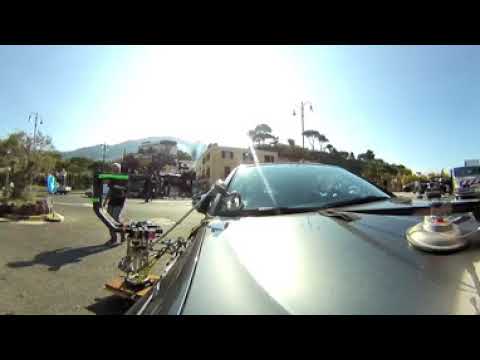The image captures the front of a car being cleaned, with the perspective taken from the level of the hood. On a bright, sunny day, the sun's glare is reflected off the windshield, partially obscuring some details. A gentleman is seen to the right of the car, casting a heavy shadow, although his specific actions are unclear. To the left of the car, there appears to be a machine or robot with a green arm, possibly engaged in polishing or washing the vehicle. The car is parked on an asphalt road, with a backdrop that includes a yellow, cube-shaped building in the center and distant trees and structures. The sky above is clear and blue, with no visible clouds. The overall scene is framed by black borders at the top and bottom of the image. The predominant colors include black, white, blue, green, light green, light blue, gray, brown, and silver.